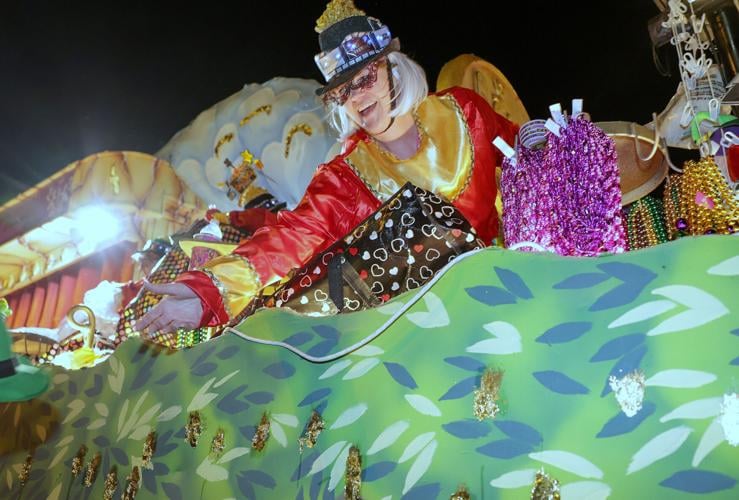In this photograph taken at a theme park parade at night, we see a vibrant and detailed scene. A woman in an elaborate costume - featuring red and gold colors, a black top hat adorned with movie reel designs and possibly card motifs, and pink butterfly glasses - leans out from a float. She has chin-length white hair and extends her right arm with a smile, seemingly tossing a golden object. The float itself is decorated with a green background that showcases light and dark blue leaf patterns, alongside gold baubles and beads. The lower part of the float, topped with a wavy design, includes white and blue leaves. Illuminated movie reels and other colorful decorations, such as purple, gold, and green beads, are visible across the float. The backdrop is a night sky, with indistinct buildings or cutouts adding depth to the festive atmosphere.